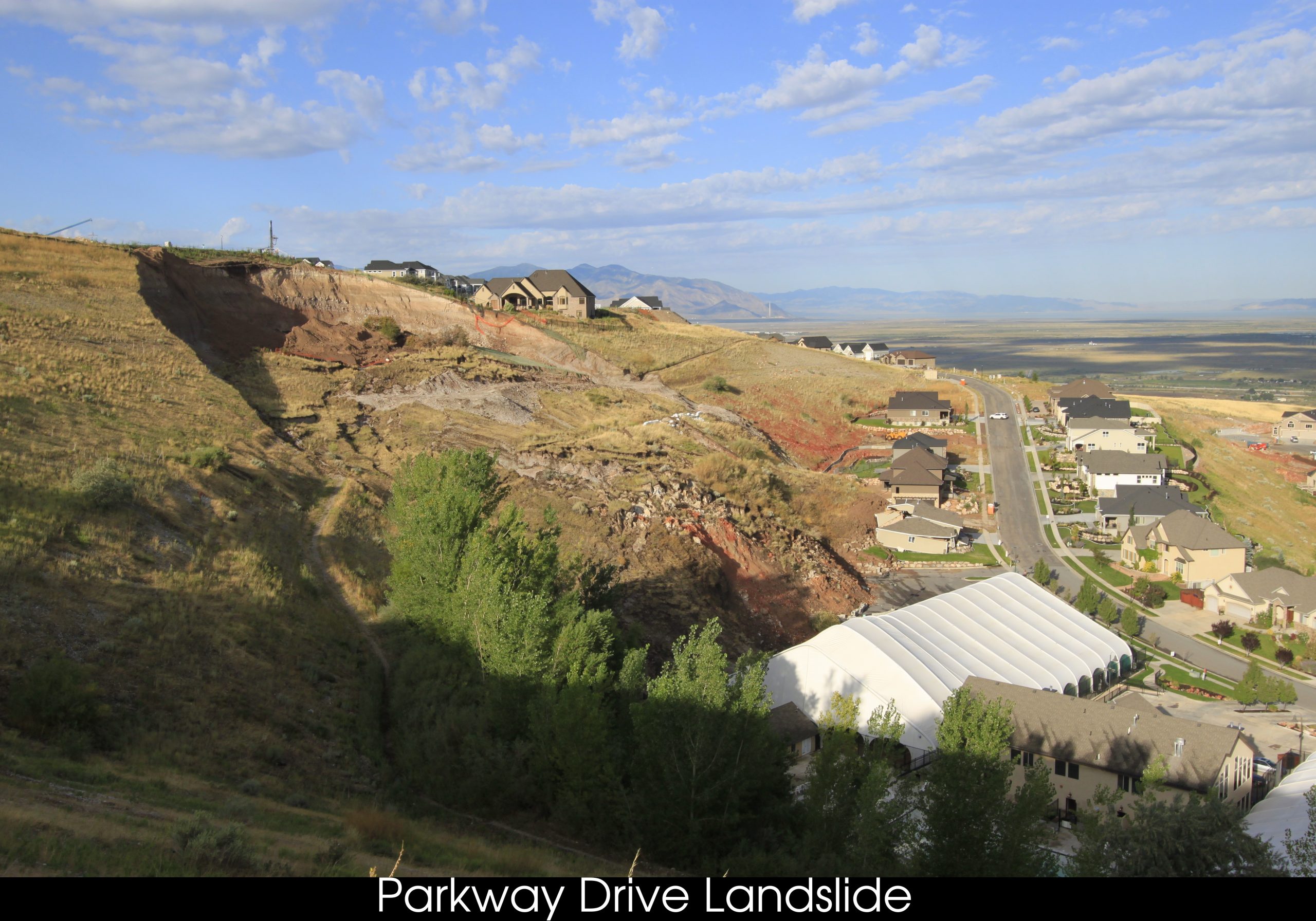The photograph showcases a bright, sunny day in a rural, hilly landscape that leads towards more mountainous terrain in the distance. In the foreground, there is a clear view from an overhead, cliffside perspective, possibly resembling a surveillance camera screenshot. The image reveals a road flanked by small structures and houses, indicating this might be a developing area with wide open spaces. A significant feature is a large, white structure, which appears to be an industrial building with a brownish-gray roof, seemingly collapsed flat on the ground, suggesting possible landslide damage. The landscape is dotted with green trees, patches of reddish soil, and light brown and green hues on what seems to be a hillside, implying the landslide's path or aftermath. The photo is labeled "Parkway Drive Landslide," underscoring the event captured. The distant background features more houses and the silhouette of mountain ranges under a blue sky with scattered white clouds, highlighting the serene yet impacted rural setting.